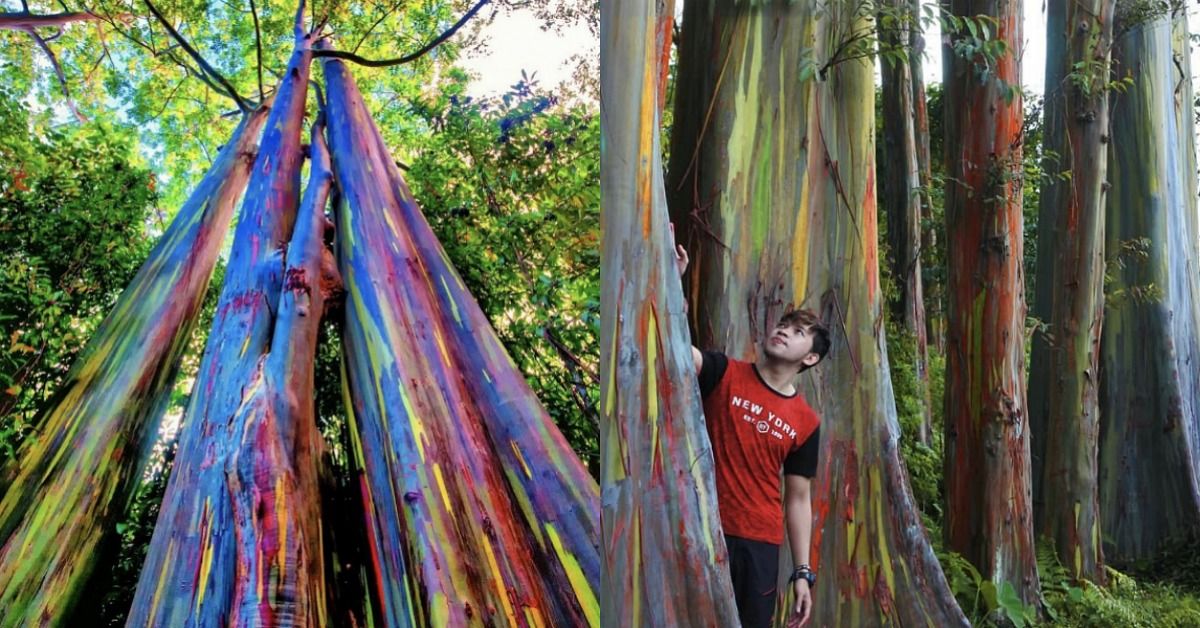The image is a composite of two photographs placed side by side. The photograph on the left captures a striking view looking upwards from the base of very tall, straight trees adorned with vibrant brushstroke patterns in blue, yellow, green, maroon, and red. These trees are surrounded by dense green foliage from neighboring trees, adding to the layered, colorful scenery. Meanwhile, the photograph on the right features a young, possibly mixed-race man—suggested to be of white and Asian descent—with dark brown hair. He is dressed in a red shirt with black sleeves and a black collar stripe, which prominently displays the word "New York" in white letters along with additional white text below it. The man, wearing dark trousers and a watch on his left wrist, stands behind one of the painted trees with his right hand resting on the trunk while he gazes upwards, immersed in the colorful forest around him.